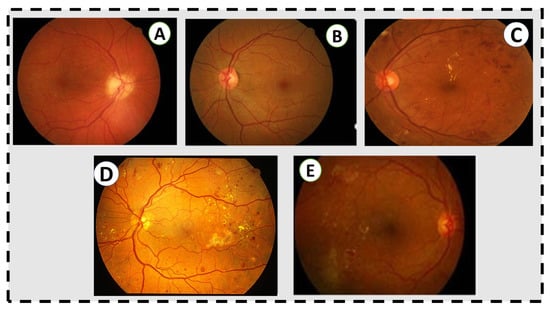The image is a detailed sequence of five photographs, each magnifying a portion of an eye, depicted on a gray background with all photos enclosed in black rectangles. These photographs are labeled with white circles containing black letters A through E. The sequence is arranged with three photographs on the top row and two larger ones on the bottom row, highlighting different angles of the eye. The eyes appear as illuminated yellow or orange marbles with intricate red veins throughout, resembling the veining one might see in an organic structure such as an embryo or the moon. Within each eye, a dark shadow or black object can be discerned, adding depth to the imagery. The predominant colors in these photographs are black, yellow, red, and white, creating a visually striking composition.